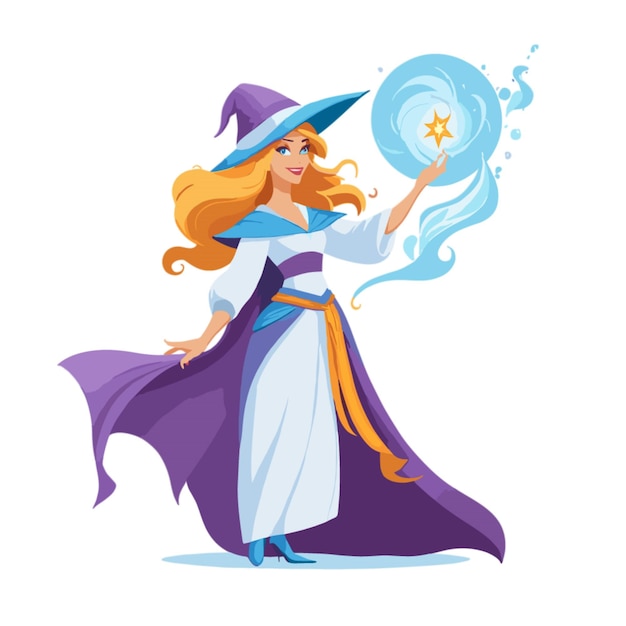This image features an animated, witch-like character with long, flowing blonde hair and pale skin, set against a completely white background. She wears a distinctive witch's hat that is teal and purple, accompanied by a flowing purple cape. Underneath, she dons a long, light blue dress cinched with a gold belt, and high-heeled blue boots. She stands in the center of the image, casting a spell with her left hand, where a star and a large sphere of water or blue flames emanate, highlighting her magical prowess. Her eyes are blue, with one being noticeably cross-eyed. This detailed rendering combines elements that evoke a cartoon or comic style, reminiscent of a Disney character.